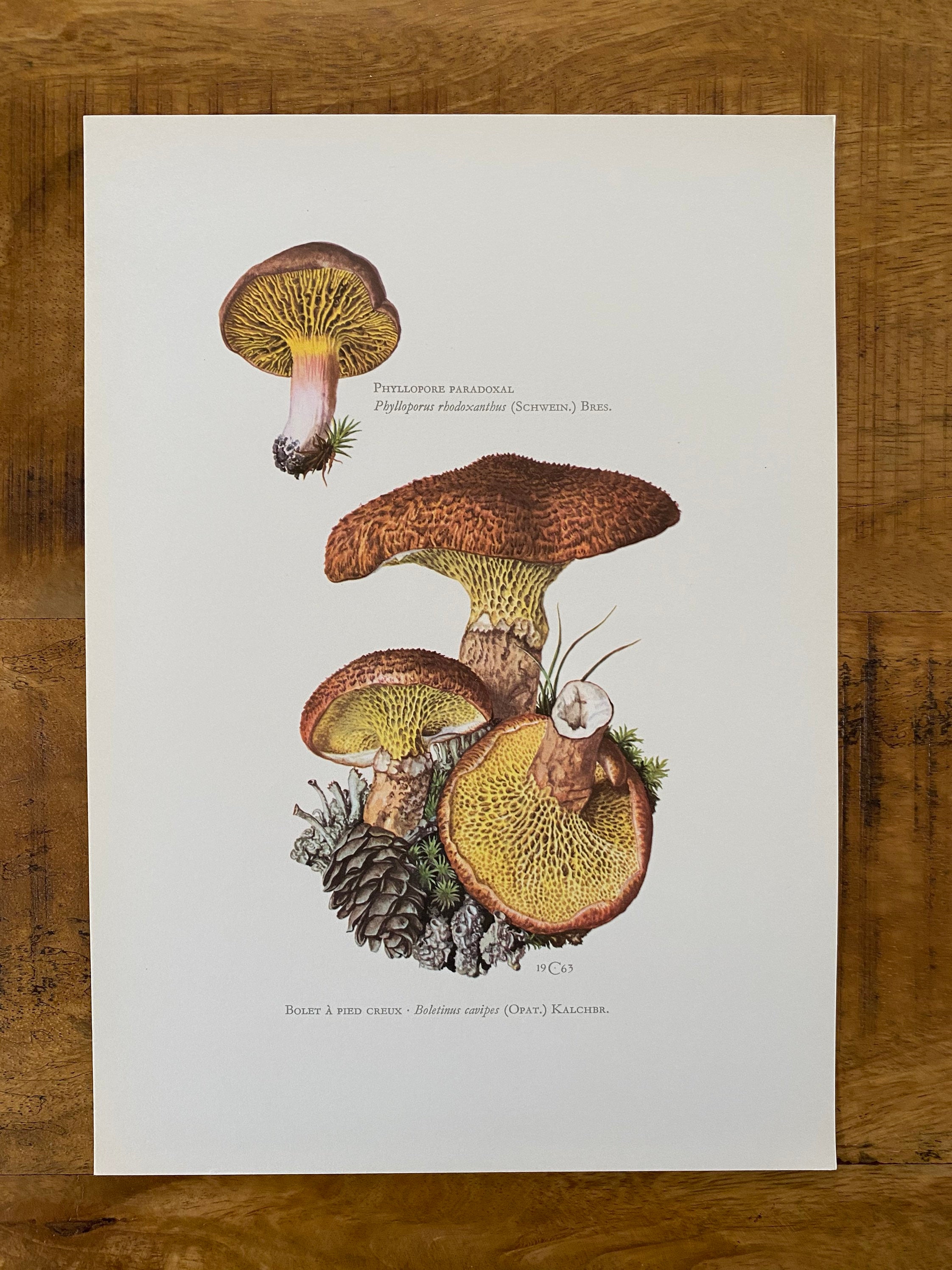The image shows a vertically rectangular sheet of white paper with fine, colored illustrations, placed on a wooden surface that frames it. The focus of the artwork is on detailed depictions of mushrooms and a pine cone. In the upper left corner, there is a single mushroom depicted with a brownish top, yellow gills underneath, and a white stem transitioning from yellow to red, showing dirt and a bit of grass at the base, suggesting it was recently pulled from the soil. This mushroom is labeled in small black text, difficult to read clearly, but it appears to say "Phylloporus paradoxus," along with a corresponding scientific name. Below this image, occupying the bottom center of the paper, are three similar mushrooms. Two of them are growing next to each other, and the third one is placed upside down, revealing the underside of the cap and gills. These mushrooms are situated in a bed of moss with details like a pine cone and small pieces of grass. Under this illustration, a numeric and alphabetical label, "19C63 B-O-L-E-T-A-P-I-E-D-C-R-E-U-X," is present, denoting perhaps a catalog or identification number.